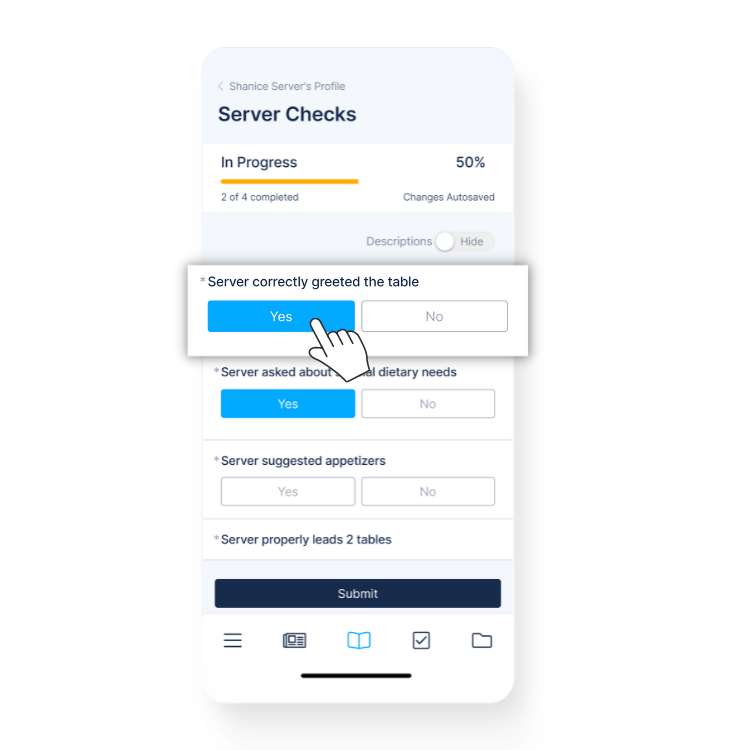The image features a user interface designed for server profile management. At the top of the interface, there's a light gray box containing blue text that reads "Shanice Server Profile," with an arrow pointing to the left. Beneath this, the section labeled "Server Checks" includes a white subsection marked "In Progress," accompanied by a yellow horizontal line and a status indicating "Two of four completed" with a progress percentage of 50%. The text also notes that changes are auto-saved.

Below this section, a gray area titled "Descriptions" is present. To its right is a grayed-out toggle bar, switched to the left in the "Hide" position. 

Further down, there is a button labeled "Server correctly greeted the table," accompanied by two options: a blue "Yes" button on the left and a white "No" button on the right. A gloved hand is hovering over the "Yes" button. Immediately below this, another prompt reads "Server asked about dietary needs," with the same configuration of a blue "Yes" button on the left and a white "No" button on the right.